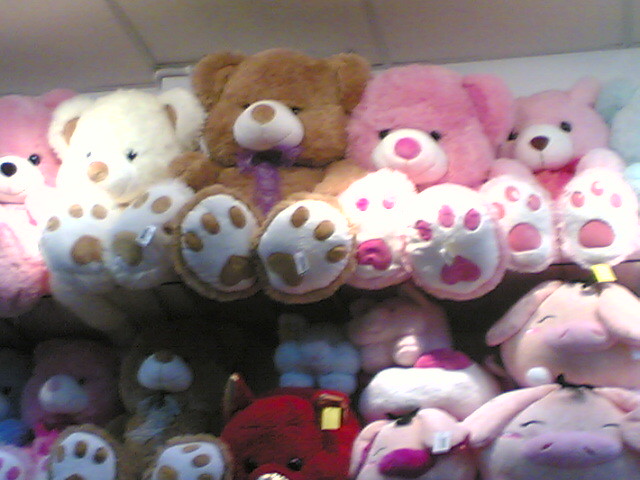The image depicts a neatly arranged display of large teddy bears and other stuffed animals against a white wall, likely in a store or display center. The top layer consists of six teddy bears lined up from left to right. The first bear is pink and white, followed by a beige-tan bear with brown feet padding, a brown and white bear with a purple ribbon around its neck, another pink and white bear, a light pink and white bear, and a blue bear that is partially cut off, showing only its head and right ear. Below this, in the shadows, is a second layer featuring fewer teddy bears and more varied stuffed animals. The second row starts with a pink teddy bear, a brown teddy bear with a light blue ribbon around its neck, followed by a red stuffed animal that resembles a bull or cow. Additionally, there are several stuffed pigs: a blue pig stacked on a pink pig, another pair of pink pigs stacked on top of each other, and a white pig in the center with a dark pink-nosed pig beside it. The display is well-lit, and the stuffed animals appear to be hanging from the wall.